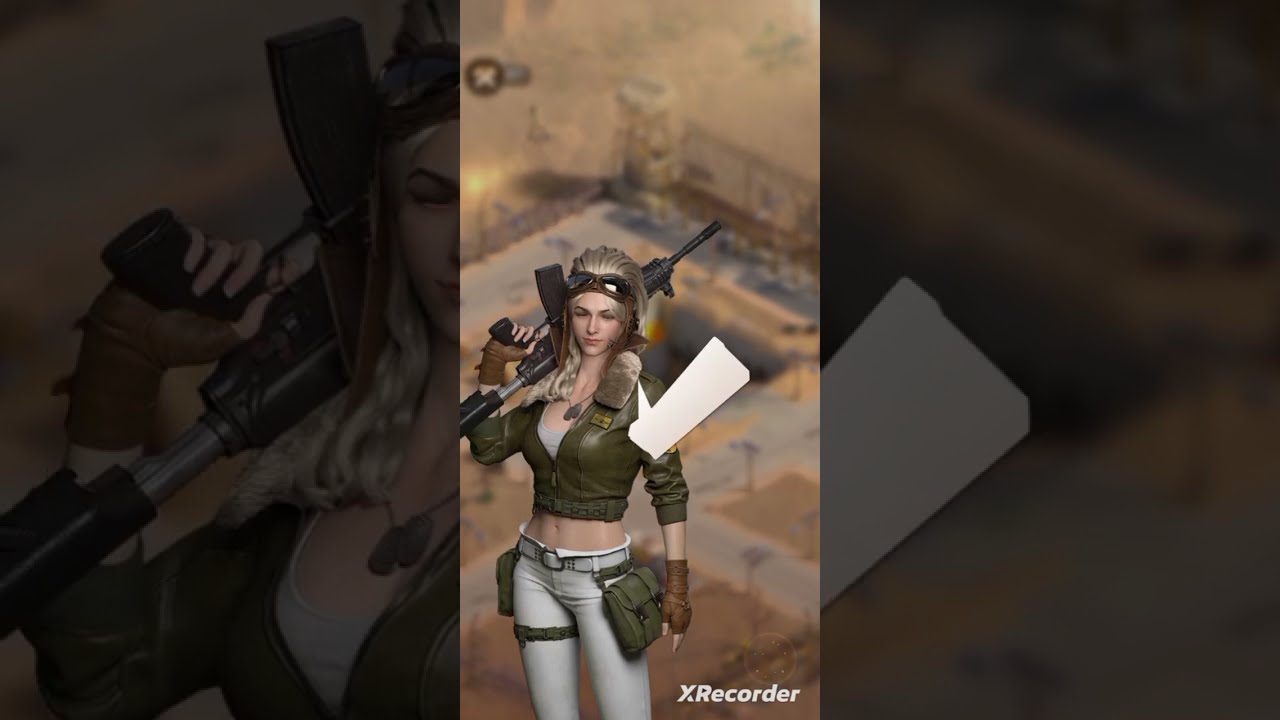In this detailed video game screenshot, the focal point is a young female character showcased in a 3D, realistic style. She stands in a slightly diagonal pose, turned towards the 7 o'clock position, seemingly gazing at the viewer. The character's outfit is a blend of military and stylish elements: a cropped army green bomber jacket with rolled-up sleeves over a white tank top, revealing her midriff and belly button. Her white, low-rise pants are accentuated with green military-style bags attached to each hip. She is equipped with brown fingerless leather gloves and aviator-style goggles resting on her forehead. Her hair is a mix of dirty blonde and gray, cascading down to her shoulders.

In her right hand, she holds a black assault rifle, possibly an AR-15, slung over her shoulder and pointed back. The character accessorizes with dog tags hanging around her neck, solidifying the military theme. The background is a bird’s-eye view of what appears to be a fortified military base in a desert environment, with sandy-colored grounds and sections cordoned off by fences and cement areas. The overall aerial perspective resembles a real-time strategy game, with a blurred-out city or compound map beneath her. Additionally, there is a blank text box near her, and the "X Recorder" watermark is visible in the bottom right corner.